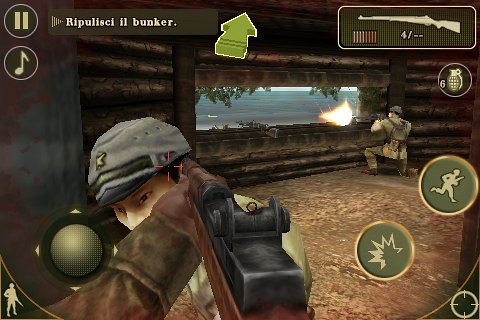In this screen grab from an unidentified video game, presented in landscape orientation, two human soldier characters are engaged in combat. The character on the left is seen in close-up, with a gun aimed directly at their head, suggesting that the player is targeting this character. The targeted character, dressed in military attire, has turned around to look over their left shoulder directly at the game player’s perspective. To the upper right of the scene, another soldier is positioned further away, shooting through an opening in a wall, hinting at a defensive stance within what appears to be a cabin or fort structure.

The screen is bordered with various interface markings and buttons that add layers to the gameplay. A green arrow suggests the direction ‘forward,’ while an adjacent button offers the option to retreat. Additional buttons include one for throwing a grenade, another to increase gun strength, and various game instructions, apparently in another language, pertaining to a bunker strategy. Also visible are buttons to pause the game and to control the game’s music, offering a comprehensive view of the game's tactical and interactive features.